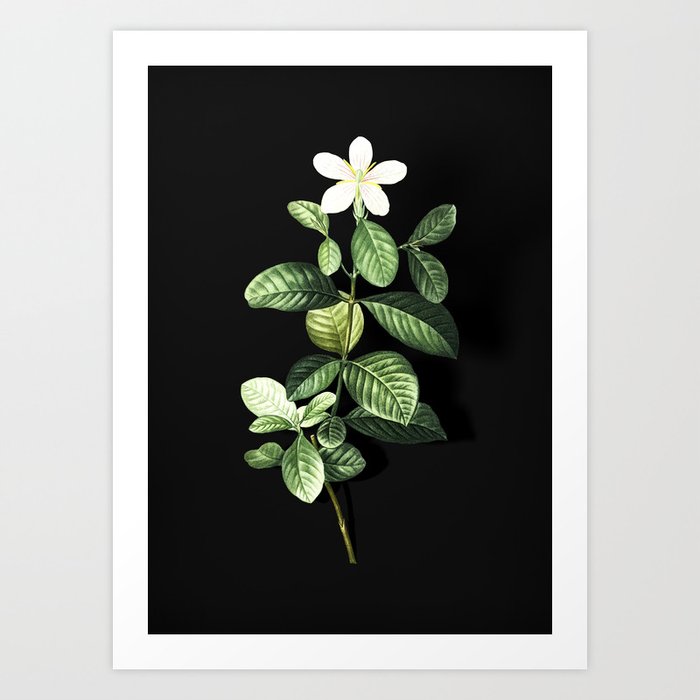This image features a highly realistic and professional piece of art framed by a thick white border, which contrasts against a plain light grey wall. The artwork itself presents a single flower with a tall, thin main stalk, adorned with numerous dark green leaves that radiate in different directions. The leaves have a slightly rubbery texture and are rendered in a shiny, almost hyper-realistic manner, standing out sharply against a pure black background. At the top of the stalk blossoms a delicate white flower with five pristine petals, accented by subtle hints of orange, pink, and yellow in the center. The overall composition is simple yet striking, combining elements of painting and drawing to create a lifelike depiction that nearly mimics a real flower.